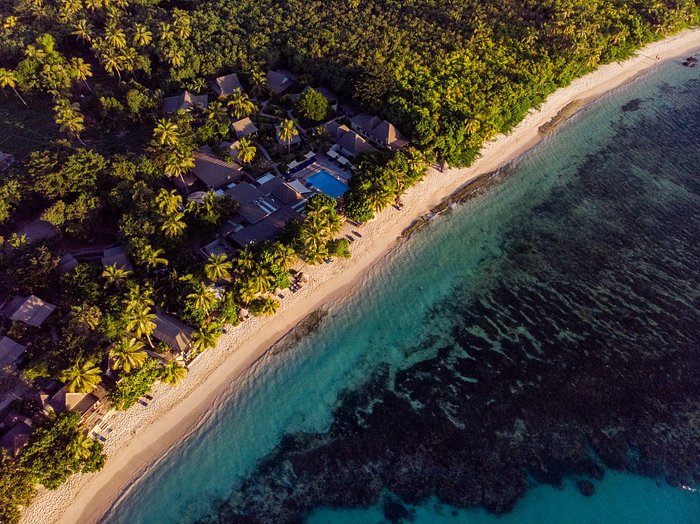This aerial view photograph, likely taken by a drone, captures a small residential area characterized by houses with predominantly brown roofs, although a few may be tan or white. The focal point of the image is a swimming pool just above the center, surrounded by lush tropical trees, including large-canopy palm trees. The scene transitions into a beach that stretches diagonally from the lower left to the upper right. Adjacent to the beach, and closer to the water, are smaller structures which are likely houses rather than hotels. The vast ocean occupies the lower right half of the image, with the water color shifting from a teal green near the shore to a dark, almost black blue in deeper sections. This gradient is punctuated by numerous dark spots on the ocean floor, possibly indicating the presence of algae or underwater growth. The sandy beach appears deserted, devoid of people or beach chairs, emphasizing the natural tranquility of the landscape.